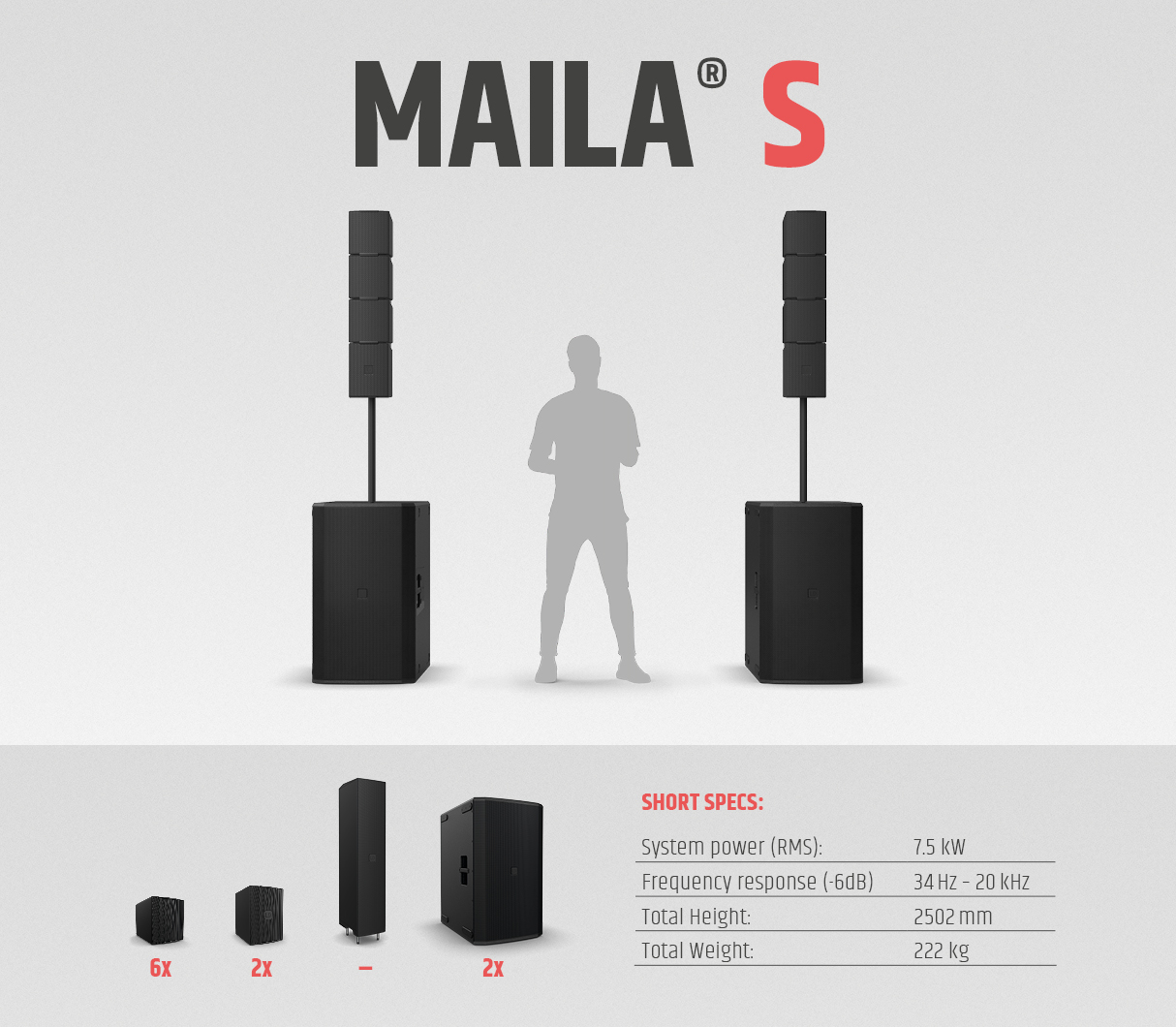The image features a promotional ad set against a light gray background. Dominating the upper two-thirds of the composition are two tall speaker towers, each about two and a half feet in height, topped with an additional section supported by a vertical pole, forming a stack of four smaller speaker units in a tall rectangular configuration. Positioned symmetrically on the left and right of a gray silhouette of a man, these speaker towers flank the central figure. The top of the ad prominently displays the brand name "MAYLA" in big black letters, immediately followed by a large red "S." Below this central graphic, the bottom third of the image provides a detailed breakout of the speaker components. This section includes images of the various elements that construct the speaker towers, accompanied by specifications such as system power, frequency response, total height, and weight. The monochromatic scheme of whites, grays, and blacks is punctuated by red text, enhancing the sleek and technical appeal of the advertisement, which appears designed for a magazine or digital platform targeting audio equipment enthusiasts.